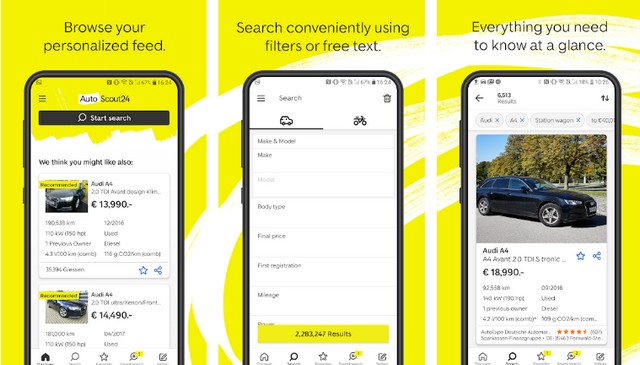This image is an advertisement for the AutoScout24 app, elegantly showcasing its main features through three distinct yellow rectangular sections displayed side-by-side.

- The first section highlights the personalized feed feature. At the top, the text reads "Browse your personalized feed." Below that, a phone mock-up displays the AutoScout24 app with a black search button prominently under the app's header. The screen beneath the button shows a section labeled "We think you might like also" with two car listings, including images on the left and their prices on the right.

- The middle section emphasizes the app's convenient search functionality. The heading states "Search conveniently using filters or free text." The accompanying phone mock-up features a search bar at the top, followed by two tabs - one with a car icon and another with a bicycle icon, indicating different search categories.

- The final section underscores the app's comprehensive listing details, with the heading "Everything you need to know at a glance." The phone screen shows a detailed car listing, specifically an Audi A4 priced at 18,990 Euros, with the car image at the top and detailed information below.

This detailed advertisement effectively communicates the app's user-friendly design and essential features, promising an enhanced car browsing experience.